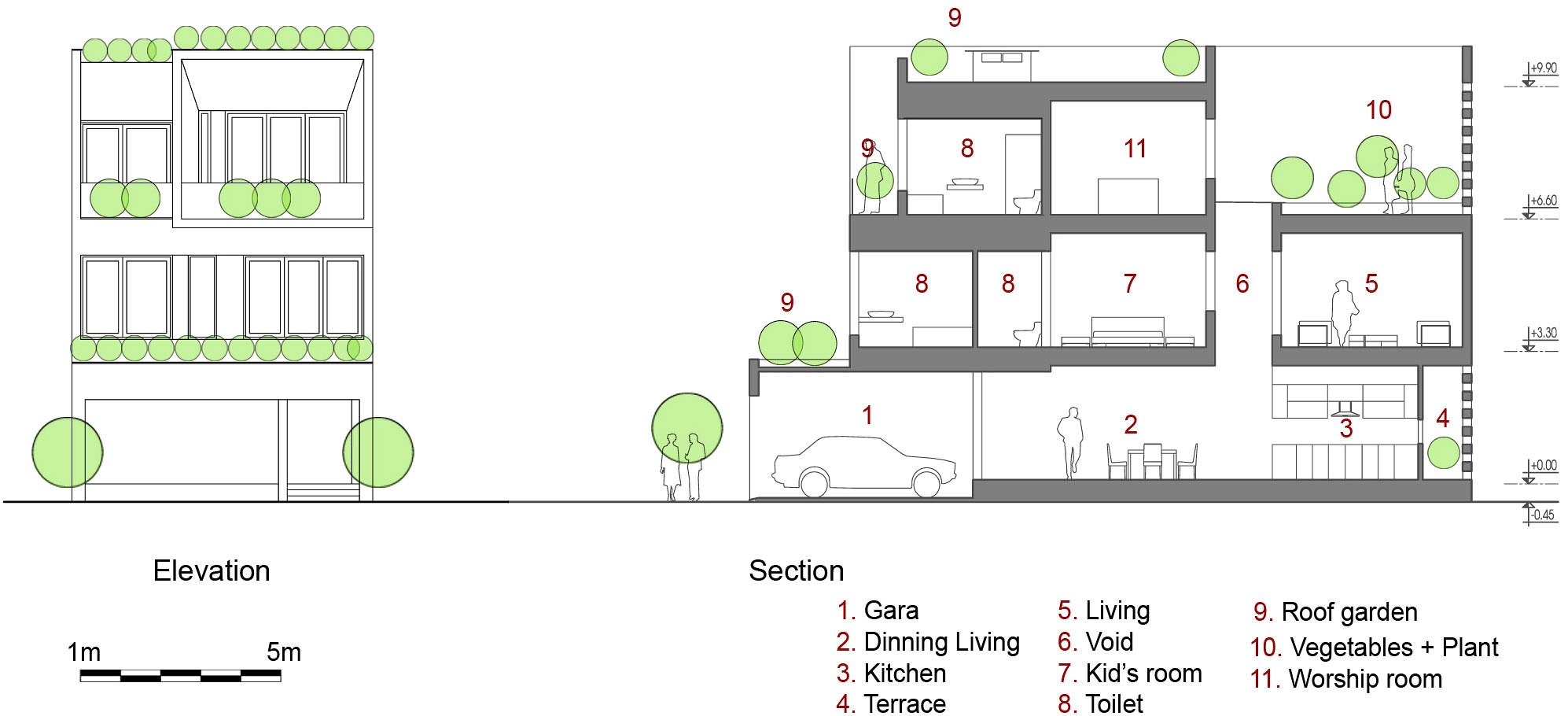The image depicts a detailed blueprint of a three-story building, showcasing both exterior and interior layouts. On the left-hand side, there is an exterior elevation illustration of the building, which includes a garage at the ground level, followed by two more floors above. The sketch is minimalist, utilizing straight lines without intricate details, but it does include tiny figures to provide a sense of scale. Green circles are scattered throughout the image, indicating specific points of interest, approximately twelve on the very top floor. 

On the right-hand side of the blueprint, a cross-sectional view of the house is presented, displaying the interior configurations and labeled numerical references. The first floor features a garage with a visible car and space for a dining room and kitchen right next to it. Moving up to the second floor, there is a roof garden above the garage, accompanied by a living area, a bathroom, and a child's bedroom. The top floor features additional space for vegetation and a worship room. Two balconies adorn the exterior; one on the second floor with two floor-to-ceiling windows, and another on the third floor with four such windows.

A legend at the bottom left provides a scale indicator ranging from one to five meters. Overall, each area within the house is meticulously labeled, highlighting areas such as the garage, dining room, kitchen, and terrace. This detailed blueprint appears to represent a multi-functional building possibly designed for communal use or worship rather than a standard residence, as evidenced by the prominent garden and worship areas.